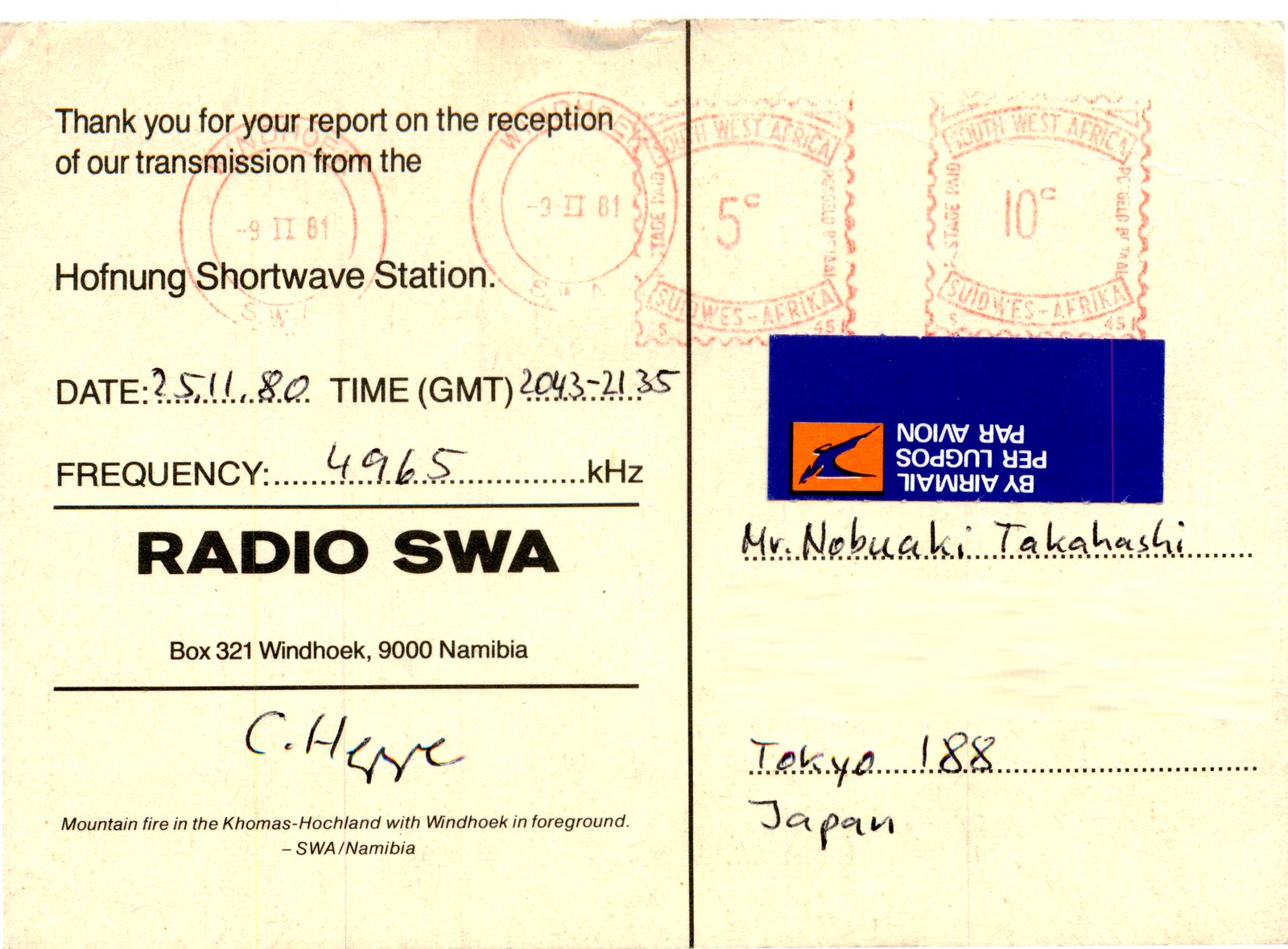The image depicts the back of a landscape-oriented, off-white beige postcard adorned with detailed print and handwritten elements. In the top left corner, the postcard features printed black text: "Thank you for your report on the reception of our transmission from the Hoth Noon Shortwave Station." Below this text are handwritten lines specifying the date as "2511.80," the time as "2043-2135 GMT," and the frequency as "4965 kHz." Further down in bold, black type, it reads "Radio SWA, Box 21, Windhoek, 9000, Namibia." Underneath is a signature followed by the caption, "Mountain Fire in the Komas Hochland with Windhoek in foreground. SWA/Namibia." A blue and orange sticker indicating "Par Avion, Per Luft Post, and by airmail" is located beneath the text. On the right-hand side, the recipient's details are handwritten: "Mr. Nobuaki Takahashi, Tokyo 188, Japan," just below several faded, red postal stamps marked "5 cents" and "10 cents," along with other symbols and postmarks.